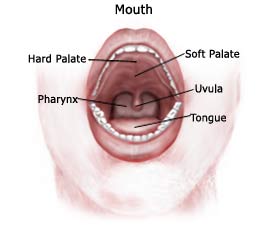This is a detailed illustration of a person’s open mouth, focusing on anatomical features. The image shows the lower part of the face, including pink-red lips, white teeth, and interior mouth structures, colored in varying shades of red and off-white. Clearly labeled in black text, lines point to specific parts of the mouth: the mouth itself, hard palate, soft palate, uvula, tongue, and pharynx. The diagram depicts the mouth open wide, revealing the tongue positioned towards the back, the tonsils, and the soft palate. The labels provide a clear, educational overview of the mouth's anatomy, illustrating its key components with precision. The illustration seems to be a digitally created diagram aimed at showcasing and identifying the vital parts of the human mouth.